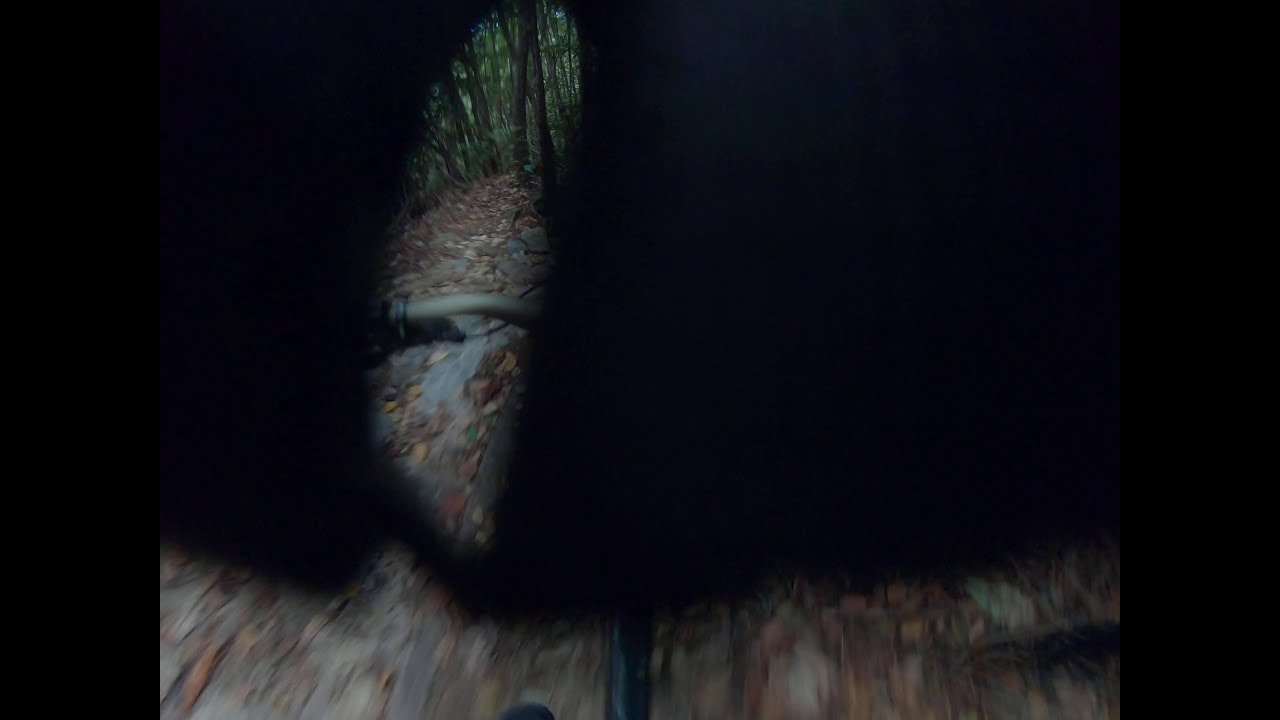The rectangular image, approximately three inches tall and six inches wide, features a photograph taken outdoors during the daytime with much of it obscured by a helmet or similar object. The left and right sides of the image are bordered with black vertical stripes, each about three-quarters of an inch to an inch wide. The shadow from the helmet covers a significant portion of the photo, leaving only an oval-shaped sliver through which the scene is visible. The bottom inch of the photograph captures a blurry view of a ground filled with dead leaves in hues of orange and black, along with some stones. A black metal pole, likely part of the bicycle's assembly, runs vertically through the center. To the left of this pole, the left handlebar of the bike is faintly visible. The camera's constrained view reveals a trail meandering forward with trees and lush green leaves in the background, indicative of a hardwood forest.